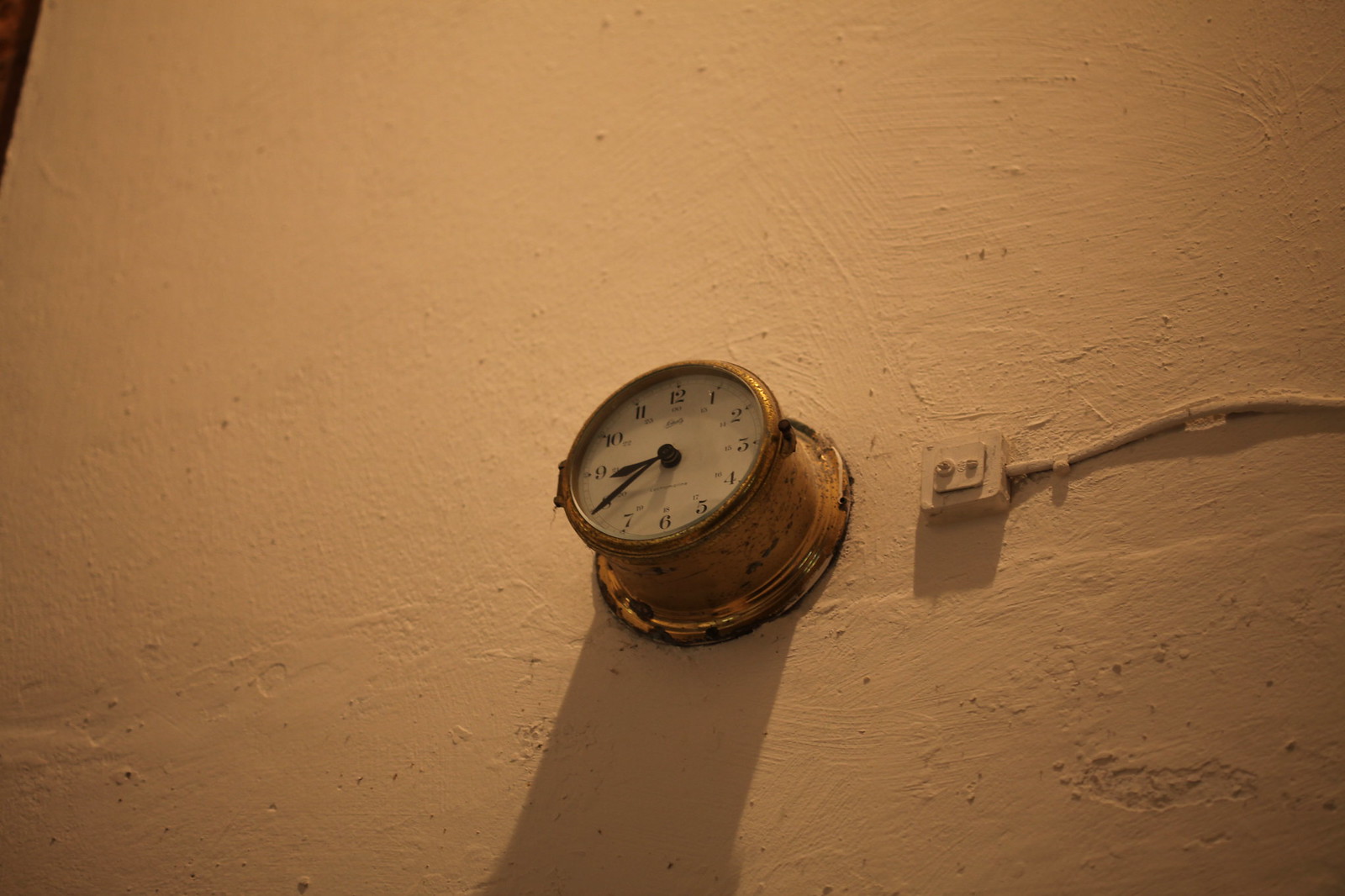The photograph captures a brass-finished cylindrical clock mounted on a beige stucco-textured wall. The clock features a round rim and an extended brass-colored lip encasing a white face with black numerals. Currently displaying the time as 8:40, the clock's pitted casing adds a touch of character. Below the clock, a small, painted-to-match beige electrical outlet and cord blend into the wall. To the side, a dark brown element, possibly a border or piece of furniture, adds contrast to the scene.